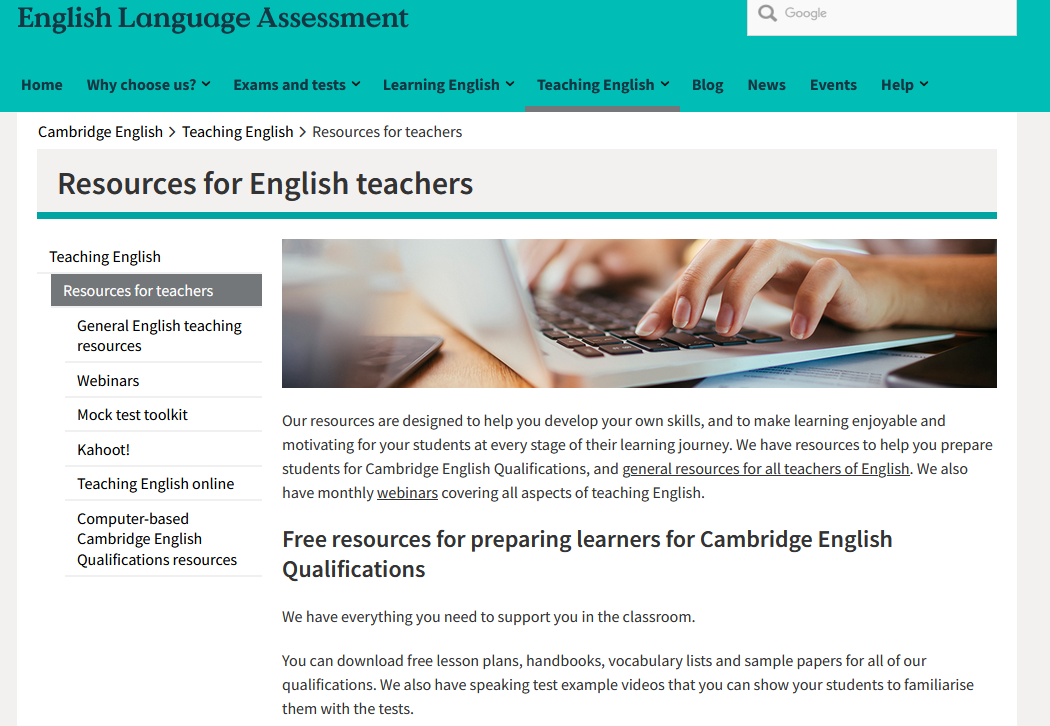**Descriptive Caption:**

The website interface features a top navigation bar in a distinct teal green color with the heading "English Language Assessment." A Google search function is embedded within this bar for easy access. Directly beneath, a black-text menu spans the page with options: Home, Why Choose Us, Exams and Tests, Learning English, Teaching English, Blog, News, Events, and Help. Following this, set against a white background, the titles "Cambridge English" and "Teaching English: Resources for Teachers" are prominently displayed.

A horizontal grey bar labeled "Resources for English Teachers" segments the page further. On the left side, a vertical column lists categories, with "Teaching English: Resources for Teachers" highlighted. Other categories include General English Teaching Resources, Webinars, Mock Test Toolkit, Kahoot!, Teaching English Online, and Computer-Based Cambridge English Qualifications Resources.

An image on the right depicts a partial view of a laptop with hands typing on the keyboard, emphasizing practical engagement. Accompanying text states, "Free Resources for Preparing Learners for Cambridge English Qualifications," underscoring the availability of supportive materials for classroom teaching.